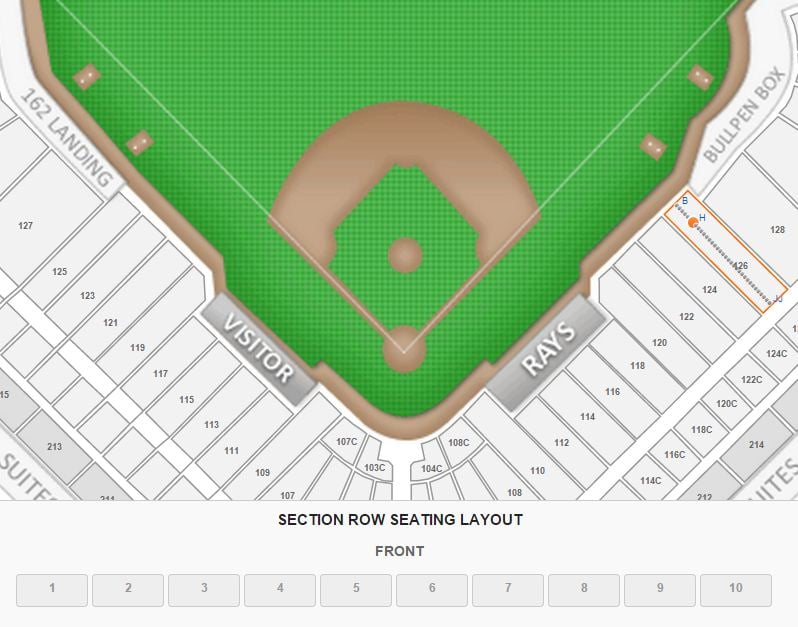This image depicts a detailed seating map centered around a baseball diamond. The diamond itself occupies the middle of the image, characterized by a lush green field with distinct white lines marking the bases and basepaths, while the infield dirt areas are rendered in brown. Surrounding the field are numerous seating sections, each meticulously numbered for easy reference.

To the left of the field, the "162 Landing" section stands out with seat numbers in the hundreds. Various designated areas, such as the "Visitor Area," "Rays Area," and "Bullpen Box," are clearly marked within the seating arrangement. Above the areas designated with numbers in the hundreds, the map transitions to sections with numbers in the 200s, which are highlighted in light gray boxes with black text for clarity.

Below the central image, the map includes an additional legend labeled "Section Row Seating Layout." This section outlines the front of each numbered section with a series of gray boxes, each representing rows 1 through 10, providing a comprehensive view of the seating organization from front to back.